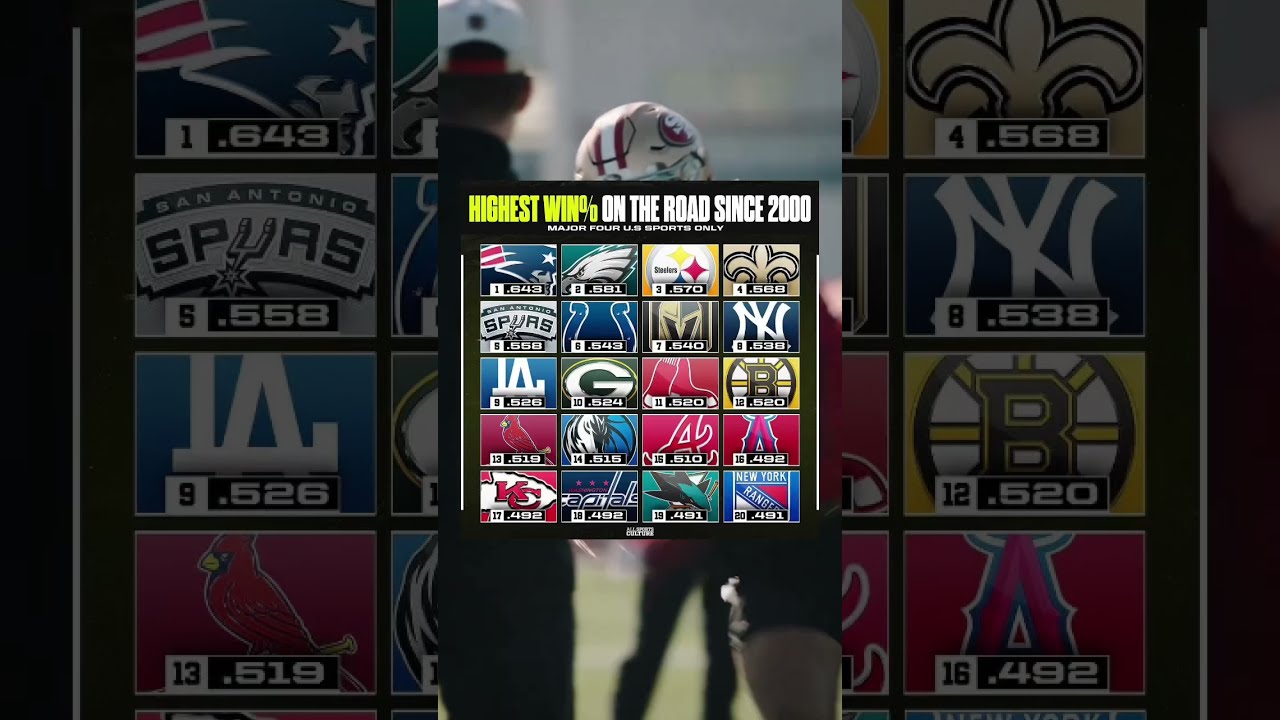The image is a horizontal rectangular informational graphic titled "Highest Win Percentage on the Road Since 2000." The background is darkened, with a partially visible football player in a helmet and a man in front of him wearing a baseball cap. On either side of them are the logos and win percentages of various major sports teams. 

On the left side, there are teams like the New England Patriots with a blue and red logo and a win percentage of .643, the San Antonio Spurs with a gray logo and .558, the LA Dodgers in white and blue with .526, and the St. Louis Cardinals in red with .519. 

On the right side, featured teams include the New Orleans Saints in gold, black, and yellow with a .568 win percentage, the New York Yankees in white and blue with .538, a team with a 'B' logo in yellow and black with .520, and another with an 'A' in red and blue with .492. 

In the center, a square displays the title, "Highest Win Percentage on the Road Since 2000," surrounded by a plethora of colorful team logos from various sports leagues such as the NFL, NBA, MLB, NHL, and others. Logos from teams like the Green Bay Packers, Kansas City Chiefs, Philadelphia Eagles, and Indianapolis Colts, among others, are also visible, all adding to the vibrant array of greens, yellows, blues, and whites.